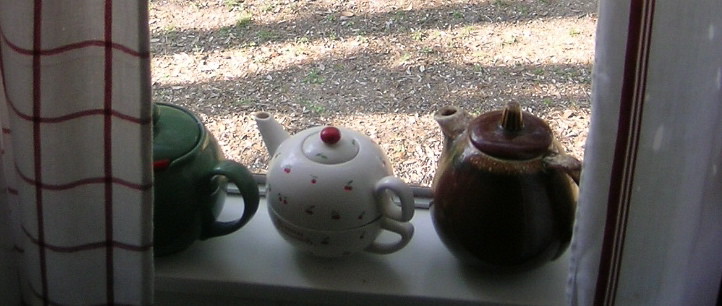This photograph features a scene viewed through a window with the focus on a windowsill adorned with three ceramic teapots. The background outside the window reveals a predominantly brown ground, dotted with dead leaves, and intersected by the long shadows cast by a couple of trees, suggesting a sparse or autumnal landscape. 

The windowsill itself is framed by two types of curtains. On the right, a white curtain with a few vertical stripes, while on the left, a curtain with a checkerboard pattern composed of large white squares intersected by thin reddish lines.

Arranged neatly on the windowsill are three distinct teapots, each facing to the left. To the far left is a green teapot partially obscured by the curtain. The middle teapot is white, roundish, and notable for its intricate design featuring two handles and a lid topped with a red knob. It also features a decorative pattern in red. On the far right sits a brown teapot that shows signs of age and wear, with a short spout completing its rustic appearance. The overall arrangement and the details of the teapots against the backdrop of the window give an impression of both charm and nostalgia.